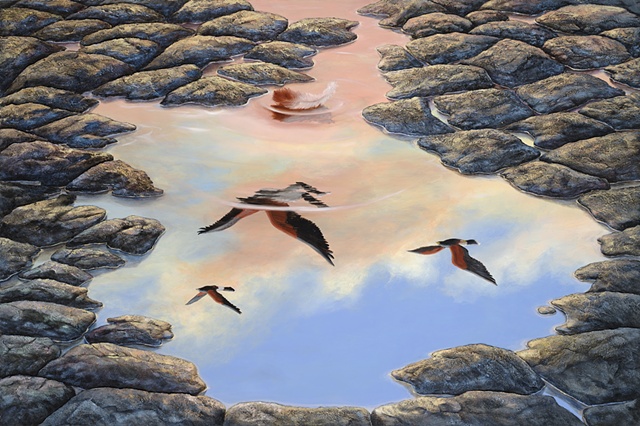This color illustration presents a realistic yet somewhat abstract perspective through a top-down view of a small body of water encircled by a border of flat, dark gray stones. In the center of the puddle, a single white and light brown feather is gently falling, causing small ripples to emanate across the smooth surface. The water reflects a serene, clear blue sky accented by lightly tinged pink and orange clouds, suggesting a sunny day. Additionally, the reflection in the puddle captures the image of three birds—possibly ducks or geese—with dark brown and black wings, dark bellies, and banded tails, soaring above. The scene is further detailed by a narrow inlet breaking through the stone border at the upper middle of the image, adding a touch of dynamic movement to the tranquil setting.